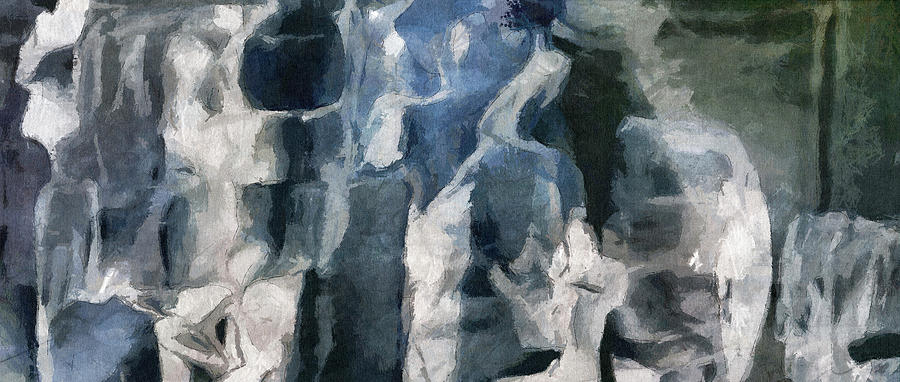This captivating image features an intricate watercolor painting that evokes the ethereal quality of swirling smoke or rugged stones. Predominantly painted in shades of gray and white, the composition also incorporates subtle hints of blue, strategically placed in the center, the top, and the bottom left of the artwork. The swirls and smears create a dynamic, almost hypnotic effect, drawing the viewer's eye across the canvas. Notably, a distinct, straight line descends in the top right corner, adding an unexpected element of structure to the otherwise fluid design.